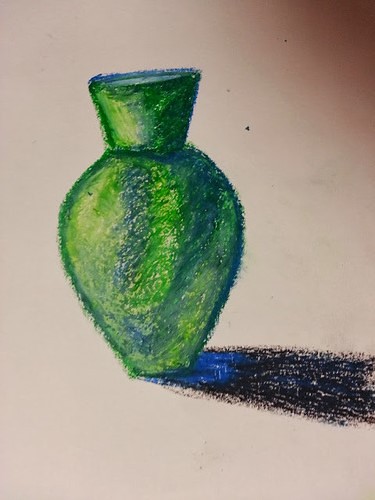The image is a photograph of an artwork featuring a vividly drawn, textured green vase that appears to be created with oil pastels or crayons on light brown paper. The vase, which becomes wider from its base and then narrows at the top before angling downward at the opening, showcases gradients of green and blue, providing a rich contrast and depth. The background transitions from a deep brownish-red in the upper right-hand corner to a very light red towards the rest of the image, adding a warm, almost soft gradient to the scene. To the right of the vase, there is a meticulously rendered shadow, beginning in a blue hue at the base and darkening into black with slightly hairy, fuzzy edges, giving it an impressionistic feel. The shadow creates an anchoring presence beneath the vase. Additionally, there is an unusual pink shadow in the top right corner, resembling a faint fingerprint or a smudge, possibly from a finger caught over the lens when the photograph was taken. This detail adds an unintended layer of curiosity to the photograph’s composition.